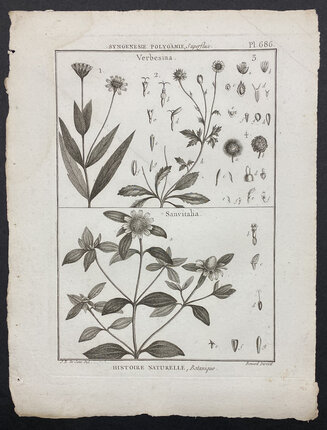This is a portrait-oriented image of a very old, worn, and possibly water-stained sheet of paper that appears to be from some sort of plant or nature guide. The paper has rough, ripped edges, and is framed by a black border. The central content is divided into two black-bordered squares, possibly ink diagrams.

At the top above the first square, faded text is partially visible, reading something like "Sugenus polygyny PL G86." Inside this upper square, we see a detailed botanical illustration labeled 'Verbena.' This illustration includes a plant with long, pointed leaves situated on the left side and a daisy-like flower. Smaller detailed parts of the plant, such as seeds and pods, are numbered and depicted on the right side.

The second lower square features another botanical illustration labeled 'Sanvitalia,' showing a plant with a central stem branching into several stems, each adorned with shorter leaves and daisy-like flowers at the top. The right side also contains smaller, numbered close-ups of the plant’s parts.

Beneath the lower panel, additional text that is hard to decipher appears, potentially saying "Histornaturale." The entire piece, with its scientific labeling and detailed plant parts, resembles an antiquated botanical drawing or guide page set against a black counter.